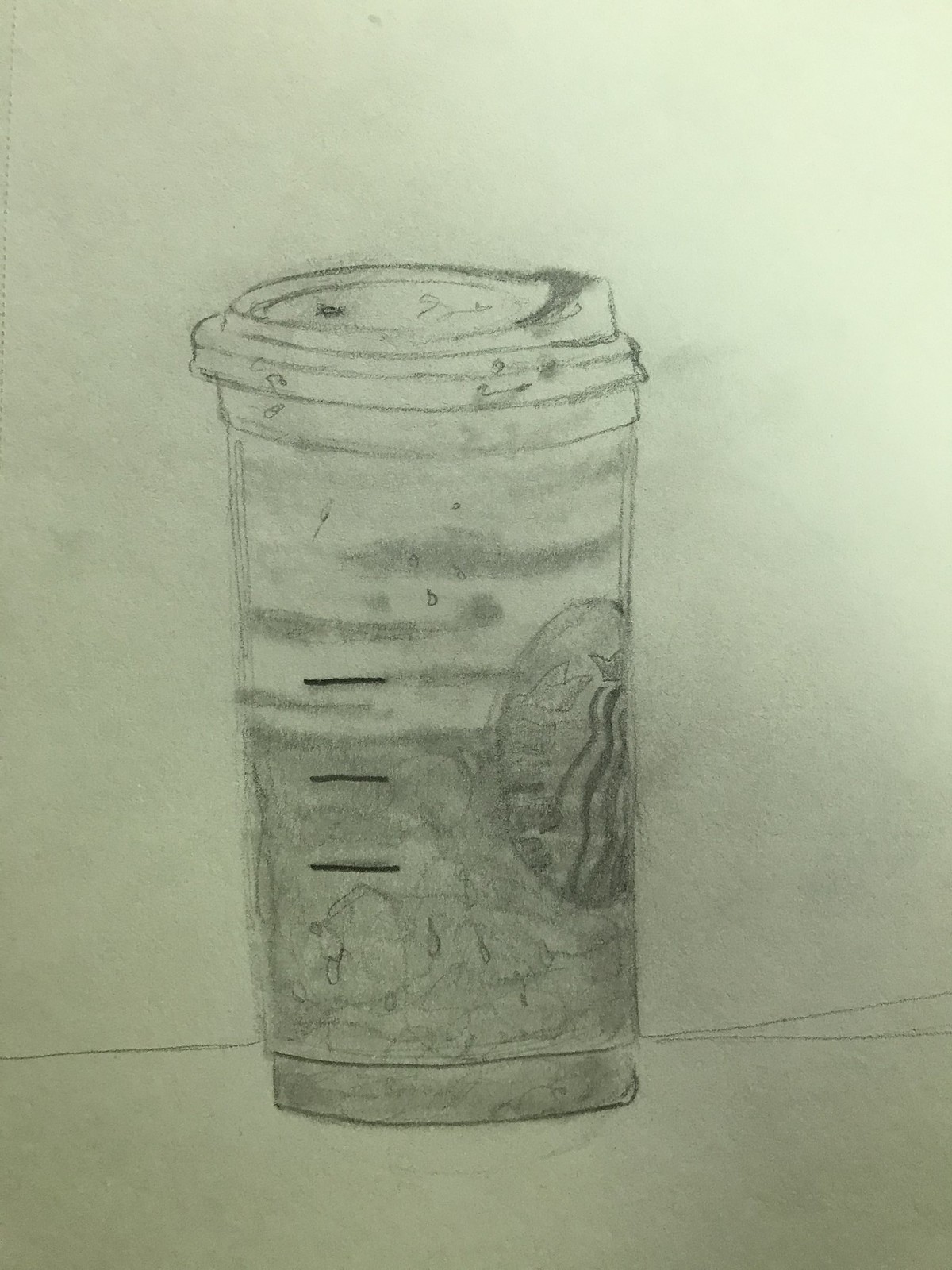The image is a black and white photograph of a pencil sketch on a white, unlined piece of paper, possibly taken from an artist's notebook. The drawing depicts a cup that closely resembles a Starbucks container. It's cylindrical with a slightly raised cap, featuring an easy-to-sip opening. The design on the cup includes part of the recognizable Starbucks logo, suggesting it might be a Starbucks cup. However, there's ambiguity as it could either be a reusable coffee cup or a paper cup with a plastic lid. The cup has intricate detailing - waves shaded in darker black towards the center and three horizontal, parallel measuring lines on the left side. This detailed shading further indicates the liquid level inside the cup.